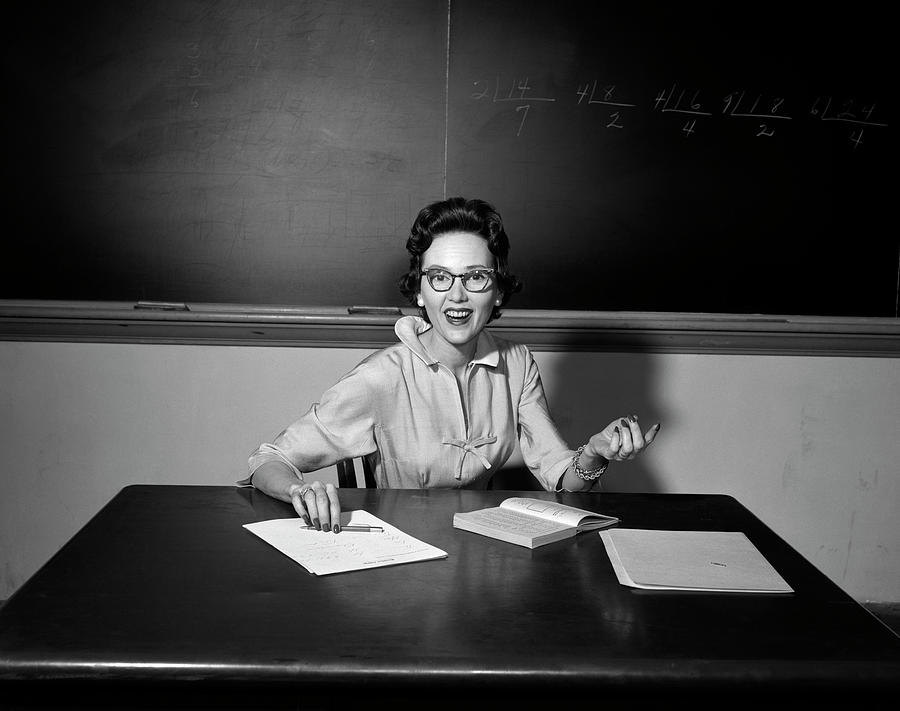A detailed black and white photo captures a poised woman seated behind a large desk in a school setting. The woman, a white female, is elegantly composed with her hair pinned back into curls and adorned with pearl earrings. She wears glasses and makeup that accentuates her features, and a bracelet graces her left wrist. She smiles warmly at the camera, as though caught mid-sentence, exuding an inviting and approachable demeanor. A plethora of teaching materials surrounds her workspace; an open book lies directly in front of her, and she holds a pen in her right hand, poised over a stack of papers. To her left, a folder filled with papers is neatly placed on the desk. Behind her, a chalkboard prominently displays math equations, partially obscured by an assortment of erasers, underscoring the academic environment. The overall scene suggests she is a dedicated teacher immersed in her educational duties.